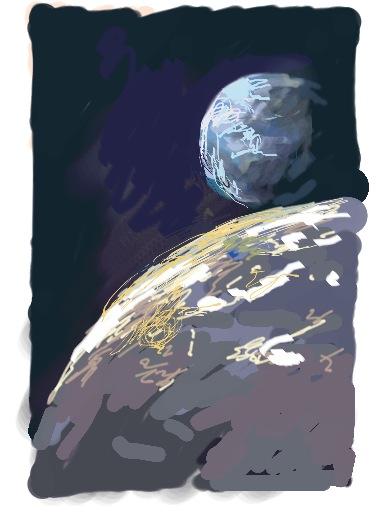In this artistic watercolor drawing, we see an evocative portrayal of a planet and its moon. The planet, depicted with a rough yet vivid brushstroke, features discernible outlines of landmasses and bodies of water. The land is adorned with white and gold squiggles, possibly representing the glow of illuminated cities or settlements, suggesting a nighttime scene. The moon, positioned in such a way that it almost appears to be touching the planet, is rendered in a gray hue with a dimpled surface, resembling lunar craters. It is further embellished with blue squiggly lines that face towards an unseen light source. This light source, implied to be off to the northwest, bathes both celestial bodies in a gentle luminosity, creating a serene and mysterious atmosphere.